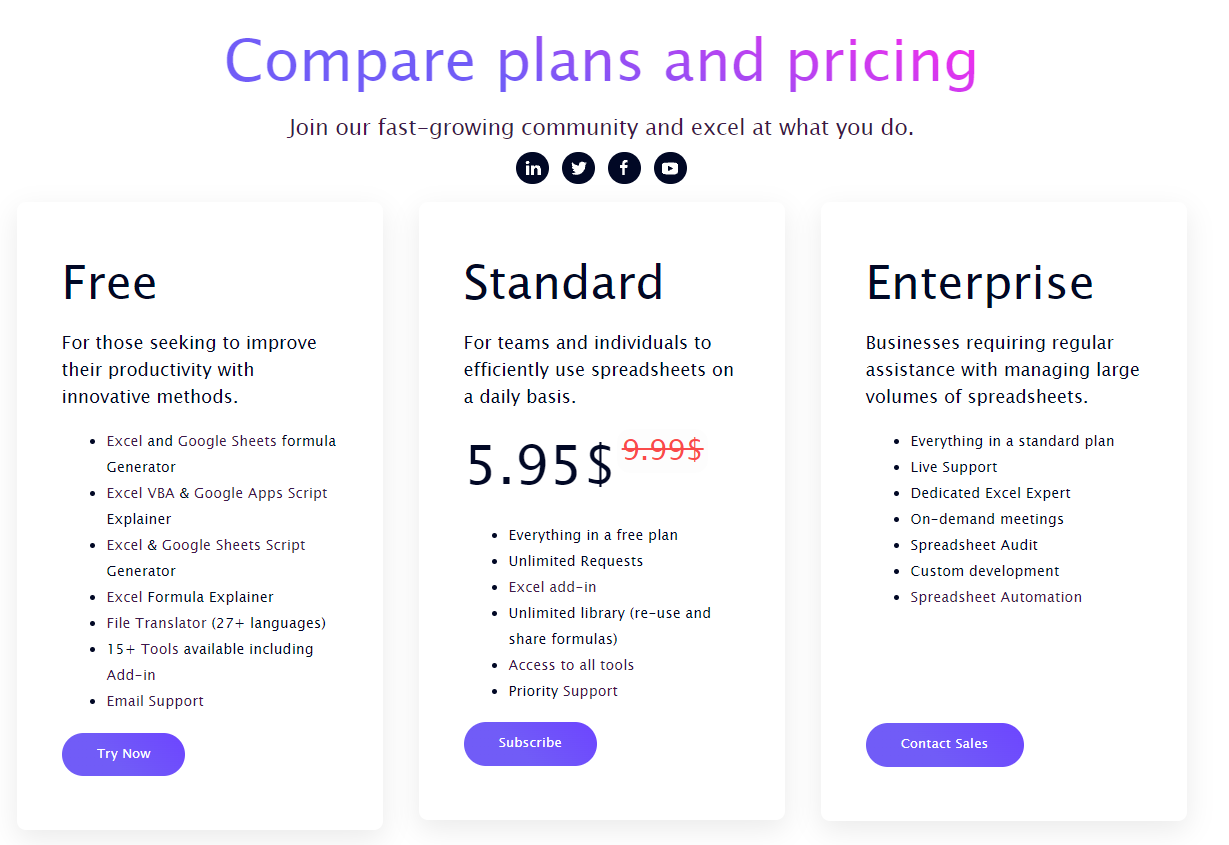### Caption:

A clean, user-friendly website screenshot with a white background, designed to capture visitors' attention at first glance. The top section features the headline "Compare Plans and Pricing" in eye-catching purple lettering. Below, a tagline in black reads, "Join our fast-growing community and excel at what you do."

Four prominent black circular icons, each hosting a white icon in the center, represent social media platforms: Indeed, Twitter, Facebook, and YouTube.

The page is structured into three vertical sections, each marked by a bold black title. The leftmost section titled "Free" caters to those seeking to enhance productivity through innovative methods. It lists multiple bullet points about features focusing on Excel, VBA, and Google Sheets, concluding with an inviting purple oval button inscribed in white text that says "Try Now."

The middle section, "Standard," is aimed at teams and individuals who use spreadsheets daily. It highlights the price "595" in bold black, while an earlier price of "999" is crossed out in red, indicating a discount. This section details additional Excel tools besides the Free plan's features, ending with a purple oval button that reads "Subscribe" in white.

The third section, titled "Enterprise," addresses businesses requiring extensive assistance with managing large volumes of spreadsheets. It elaborates on features including spreadsheet automation in a series of bullets, ending with a larger purple oval button stating "Contact Sales" in white. 

Each section is equipped with ample information designed to help users make informed decisions about the plan that best suits their needs.